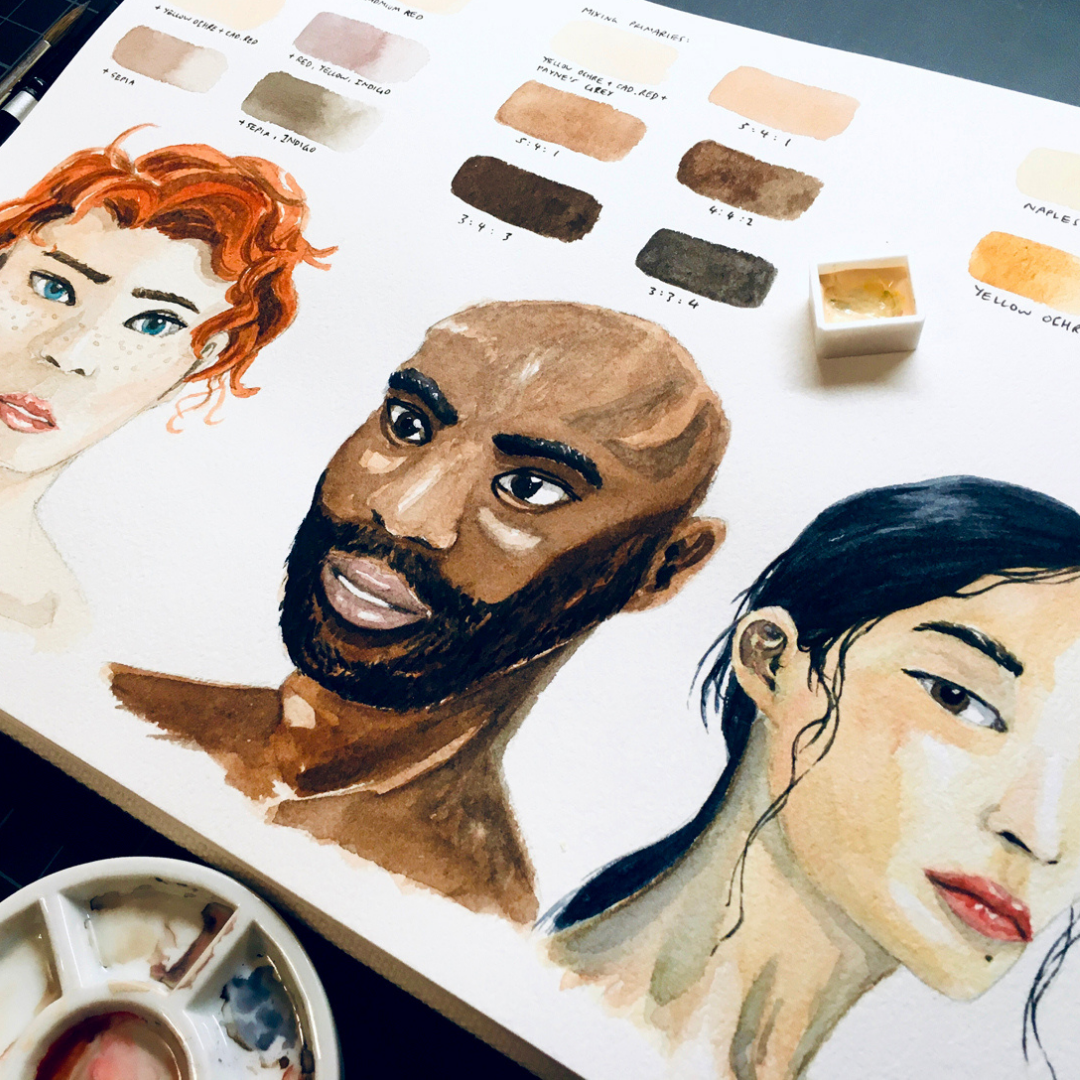This photograph captures a watercolor sketchpad featuring concept art primarily composed of three distinct head-and-shoulder illustrations. Dominating the page are the detailed busts of three individuals: on the left, a Caucasian woman with vibrant red curly hair; in the center, an African man sporting a bald head and a goatee; and on the right, an Asian woman with serene features. Along the bottom edge of the sketchpad, a series of meticulously painted skin tone swatches are laid out, likely for testing and refining colors. Above the portraits, evenly spaced rows of watercolor swatches display various hues, suggesting a methodical exploration of the watercolor paint's range and quality. The overall composition provides a glimpse into the artist's process of perfecting skin tones and experimenting with different watercolor pigments.